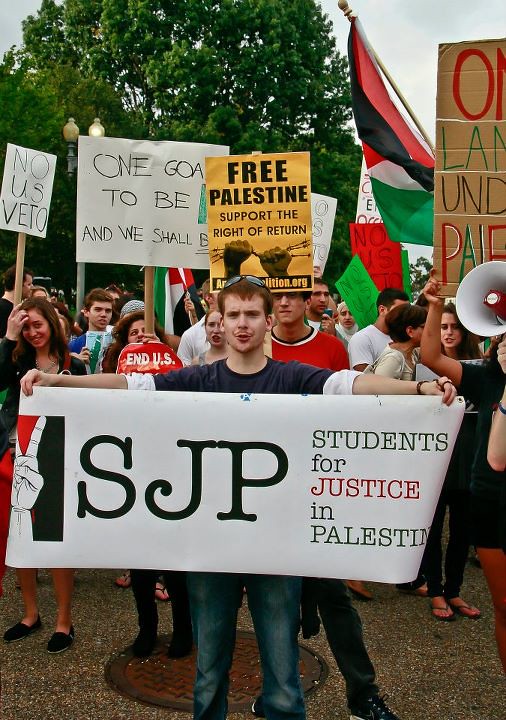In this daytime photograph, a male protester stands prominently in the center, wearing a gray long-sleeve shirt paired with blue jeans. He holds a sizable white banner with a peace sign symbol, prominently displaying the letters "SJP" for Students for Justice in Palestine. The right side of the banner details the full name of the organization. Surrounding him, a crowd of protesters carries handmade signs with messages such as “No U.S. Veto,” “Free Palestine,” and “Support the Right to Return.” Various signs and a megaphone hint at the dynamic atmosphere, with slogans in red, black, and white letters on cardboard cutouts. Notably, a flag in red, black, white, and green flutters on a brown stick, adding to the visuals of the protest. The backdrop includes green trees and a sky that appears white, framing the scene of activists standing on a gray street, united in their peaceful demonstration.